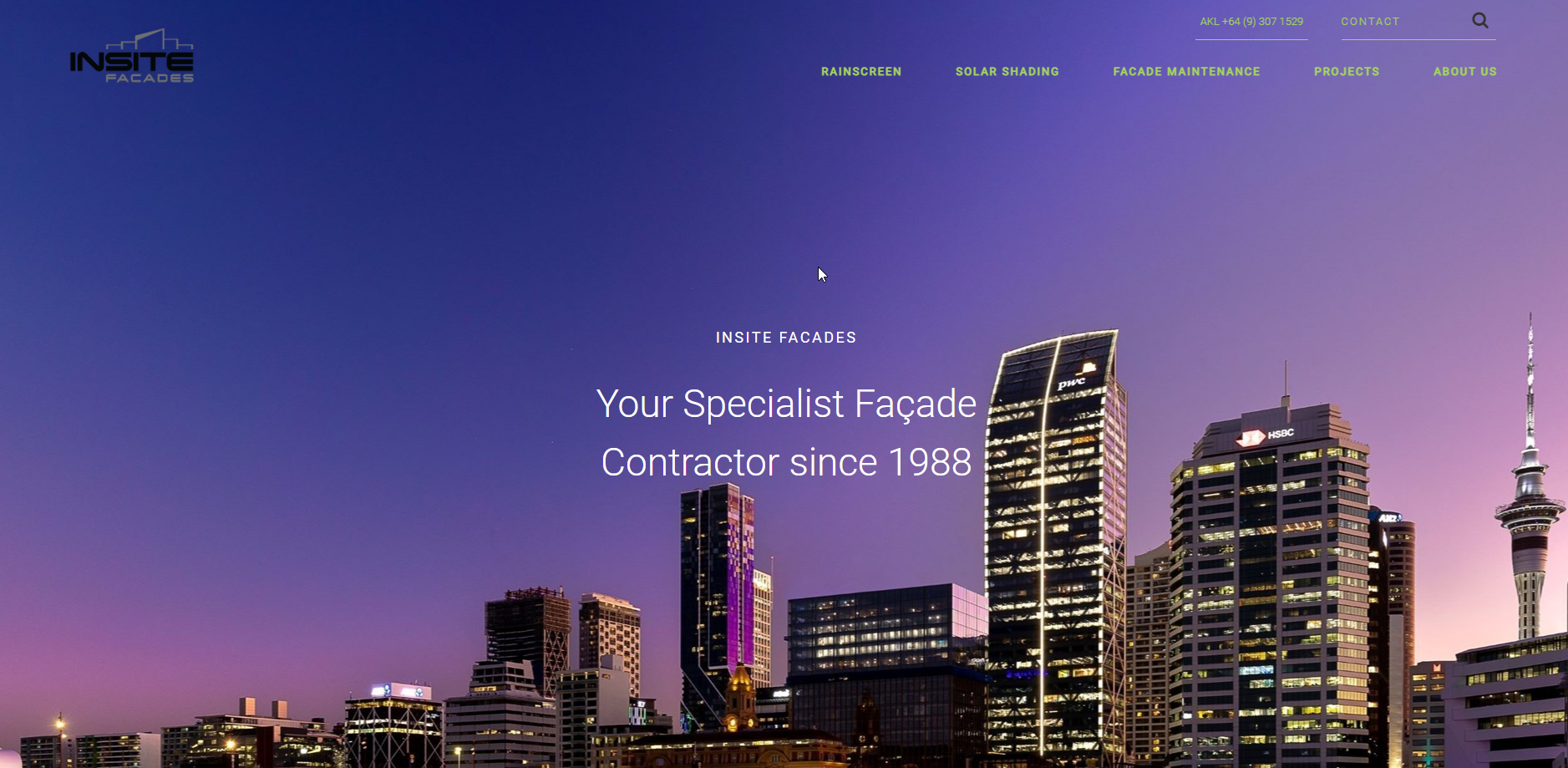This screenshot is taken from a website page of "Insight Façades." At the top, the word "INSIGHT" is prominently displayed in all capital black letters, exuding a strong presence, followed by "FACADES" in a softer, beige color. Behind the text, a cityscape with various buildings is visible, providing an urban backdrop.

On the right side of the page, there's a list in greenish print that reads: "Rain Screen," "Solar Shading," "Facade Maintenance," "Projects," and "About Us." Above this list, the website includes a phone number and a contact area for inquiries.

Centrally positioned, the image showcases a dramatic sunset sky with hues of purple, giving the scene an enchanting aura. The city buildings, some illuminated with lights, vary in height, creating a dynamic skyline. The taller buildings stand proudly, while shorter structures fill in the urban landscape.

In the center of this scenic backdrop, the company's slogan "Insight Façades" is displayed clearly. Below this, a statement reads: "Your specialist facade contractor since 1988," emphasizing their long-standing expertise in the field.